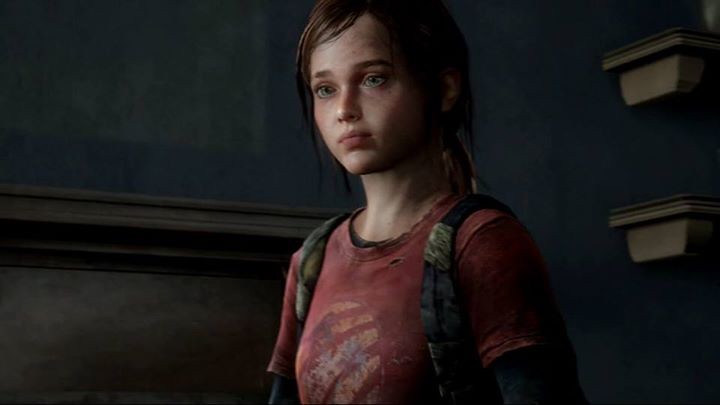A young girl with medium-length, dark blonde hair gazes thoughtfully into the distance, slightly to the left. Her expression conveys a sense of worry and sadness. She is dressed in a layered outfit, consisting of a black long-sleeve shirt beneath a red short-sleeve shirt, and appears to be carrying a backpack. Behind her is a backdrop of a dark blue wall, which constitutes the upper half of the setting. The lower portion of the wall is made of brown wood. There are also two brown rectangular protrusions on the blue surface, possibly meant for displaying ornaments.